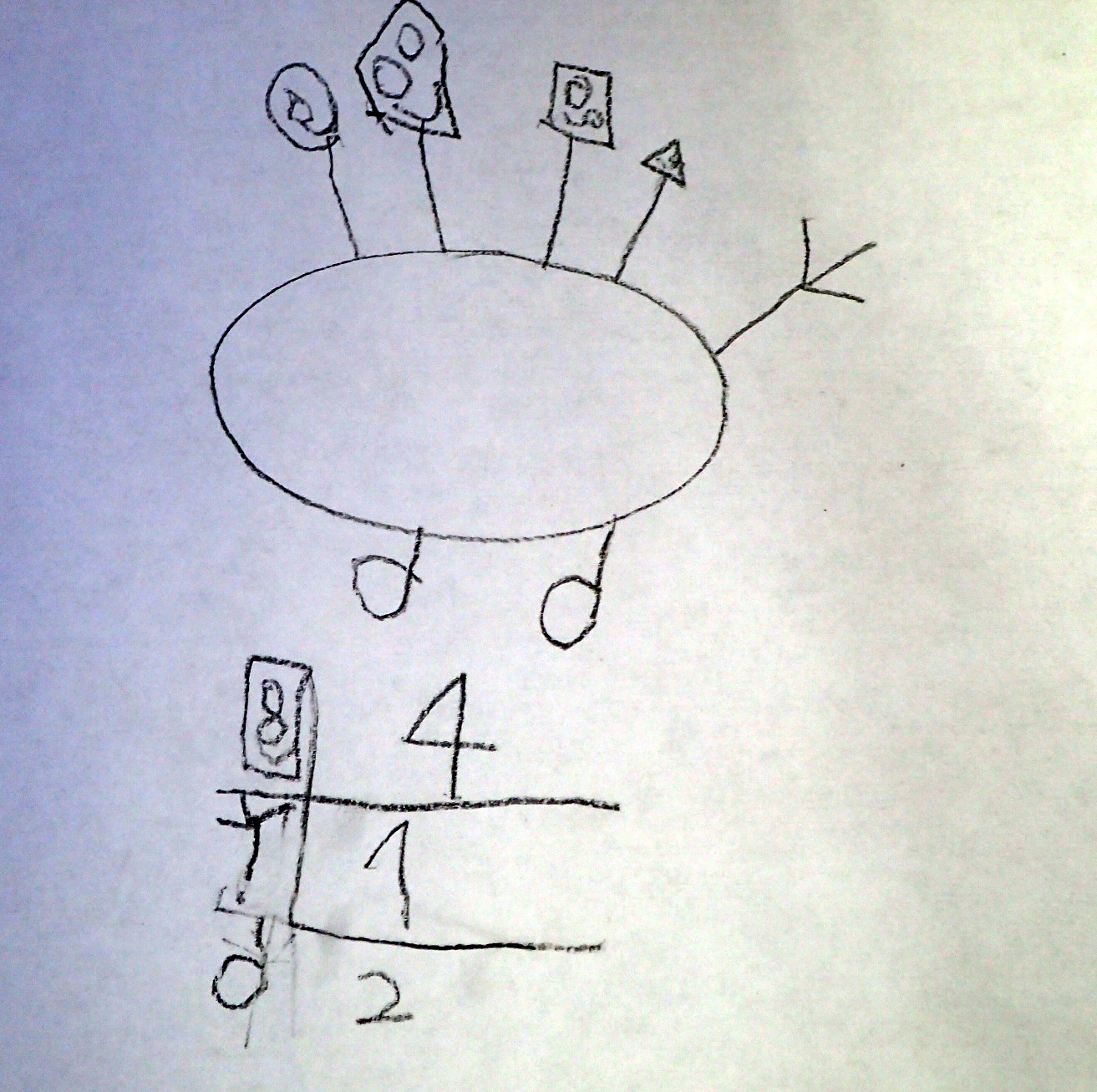A simplistic hand-drawn illustration on white paper features childlike, abstract elements rendered in what appears to be black crayon or pencil. At the top of the drawing, a roughly oval shape is adorned with what seems to be four distinct faces, though their exact nature is ambiguous. Extending from this oval form are two legs, two feet, and a single hand. Below this entity, there is a table-like structure inscribed with a series of characters that include the numbers 8, 4, 1, 2, and possibly a 0 or a lowercase 'd,' along with what might be a 7 or the letter 'T.' The entire drawing is characterized by the unrefined and whimsical style typical of a young child's artwork, leaving the rest of the paper blank and stark in contrast.